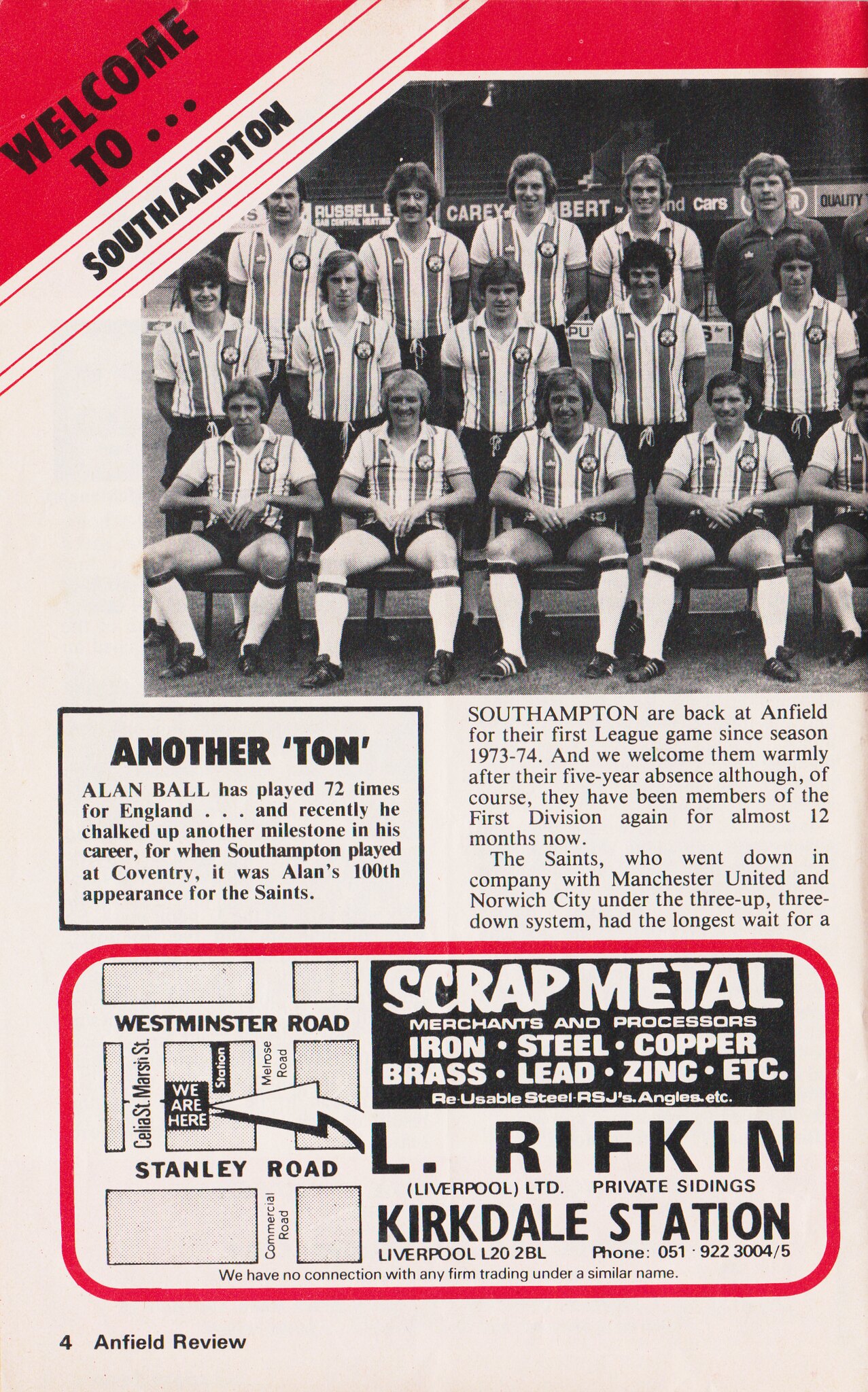The image is a detailed page from a book or magazine, featuring the welcoming headline tilted at an angle, "Welcome to Southampton." The text is highlighted with a red bar for "Welcome to" and a white bar with thin red borders for "Southampton." Dominating the upper middle section is a black-and-white team photograph of what appears to be a soccer team. The team consists of 15 players; the bottom row is seated, while the others stand. They are all dressed in identical striped uniforms, and the photograph has a bit of nostalgic charm.

Beneath the team photo is a headline, "Another Ton," enclosed within a thin black rectangle. This section contains an article with serif font providing information on Allen Ball. Adjacent to this, there's a rounded rectangle, bordered heavily in red, serving as an advertisement for a scrap metal company. This ad features a map and detailed address information, listing metals such as iron, steel, copper, brass, lead, and zinc. The advertisement mentions locations like El Ripon, Kirkdale Station, Westminster Road, and Stanley Road. The background of this page is white, with a red corner and additional red outlines enhancing the overall design.